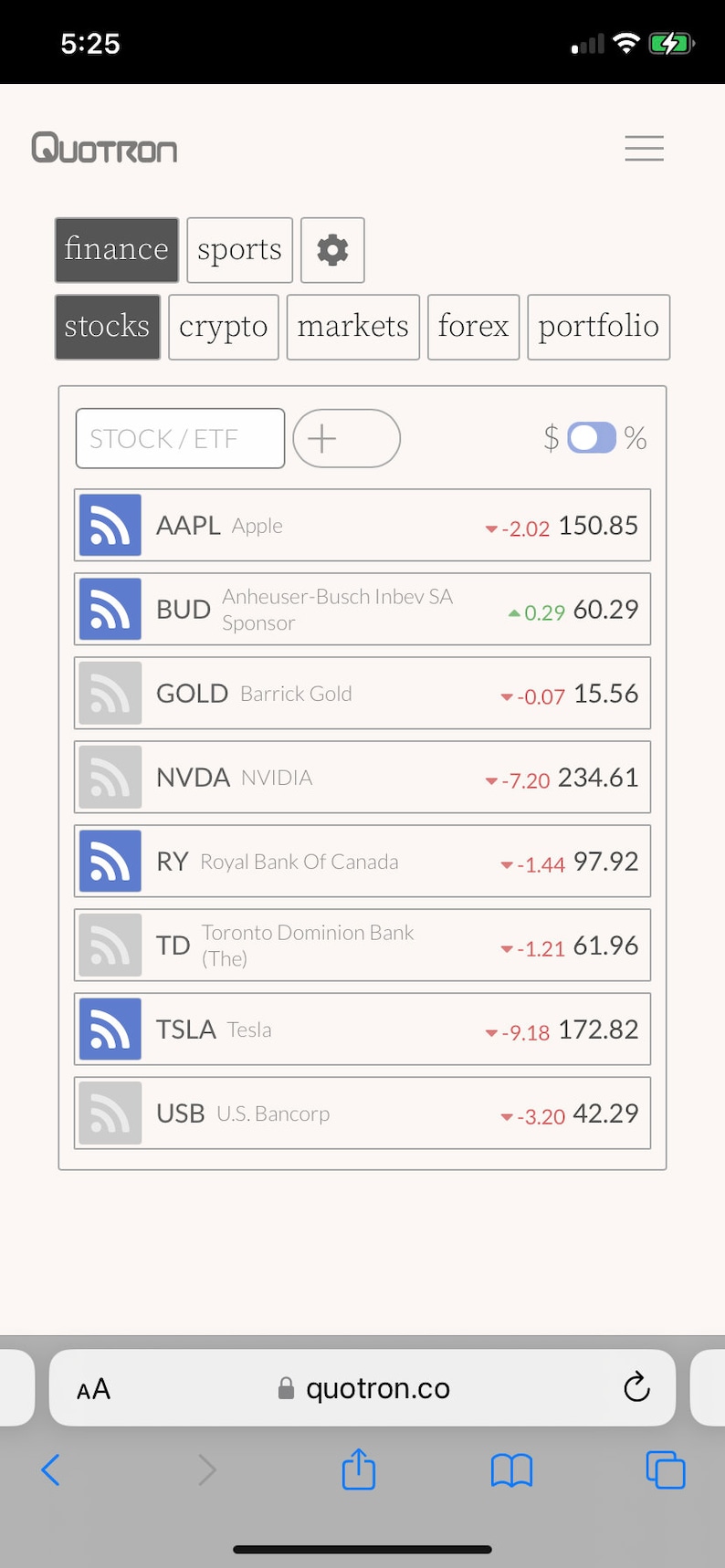The image depicts a financial monitoring screen displaying various essential details and market updates. The time shown at the top is 5:25. The signal strength icon indicates one bar, and the battery icon is visible next to it, reflecting the device's power status. The word "Quotron" is prominently displayed at the top. Beneath it, a gray-highlighted tab labeled "Finance" is selected. Adjacent to "Finance" are tabs for "Sports" and "Settings."

Further down, the screen contains several gray-highlighted categories: "Stocks," "Crypto," "Markets," "Forex," and "Portfolio." Below these categories is a white input box marked "Stock/ETF." Nearby, an oval button with a plus sign and a displayed dollar sign marked as "On" appears, followed by the number 96.

The main section of the screen lists various stock updates:

- **AAPL Apple**: Down 2.02 to 150.85.
- **BUD Anheuser-Busch SA Sponsor**: Up 0.29 to 60.29.
- **GOLD Barrick**: Down 0.07 to 15.56.
- **NVDA NVIDIA**: Down 7.20 to 234.61.
- **RAI**: Down 1.44 to 97.92.
- **TD**: Down 1.21 to 61.96.
- **TSLA Tesla**: Down 9.18 to 172.82.
- **U.S. Bancorp**: Down 3.20 to 42.29.

The overall appearance suggests a dynamic and comprehensive tool for tracking financial markets and stock performance in real time.